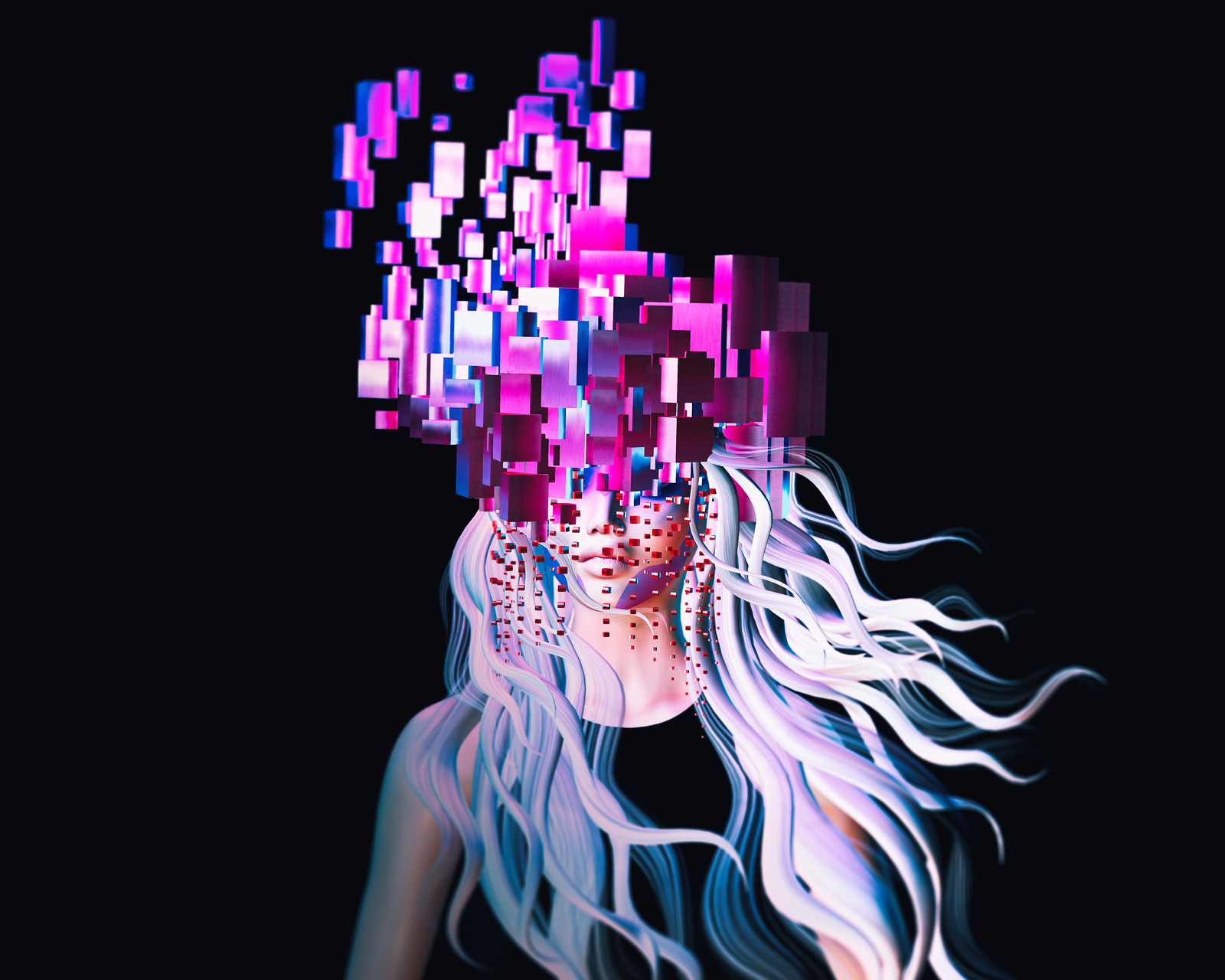This detailed computer-generated image features a young Caucasian woman with long, flowing white hair that is slightly blowing to the right of the image. She is facing the camera directly, with her arms straight at her sides, elbows slightly bent. The woman's resemblance to a character from "Game of Thrones" is evoked by her complexion and general facial structure. She is clad in a black tank top, and her overall demeanor is youthful despite her white hair.

The most striking aspect of the image is the unusual and artistic pixelation effect that begins around two-thirds up her head. The top portion of her head appears to be exploding into numerous geometric shapes and blocks in varied sizes, primarily in shades of fuchsia, but also incorporating hues like white, blue, deep purple, and crimson. These pixelated blocks seem to be floating away from the top of her head, creating a dynamic and surreal visual effect.

The background of the image is pitch black, which contrasts sharply with the woman's white hair and the colorful pixelation. The lower part of her face also has smaller pixelated disruptions, obscuring her eyes but leaving her nose and smiling mouth visible. The overall effect creates an impression of thoughts or identity being fragmented and dispersed into the digital ether, contributing to a hauntingly beautiful and thought-provoking visual composition.